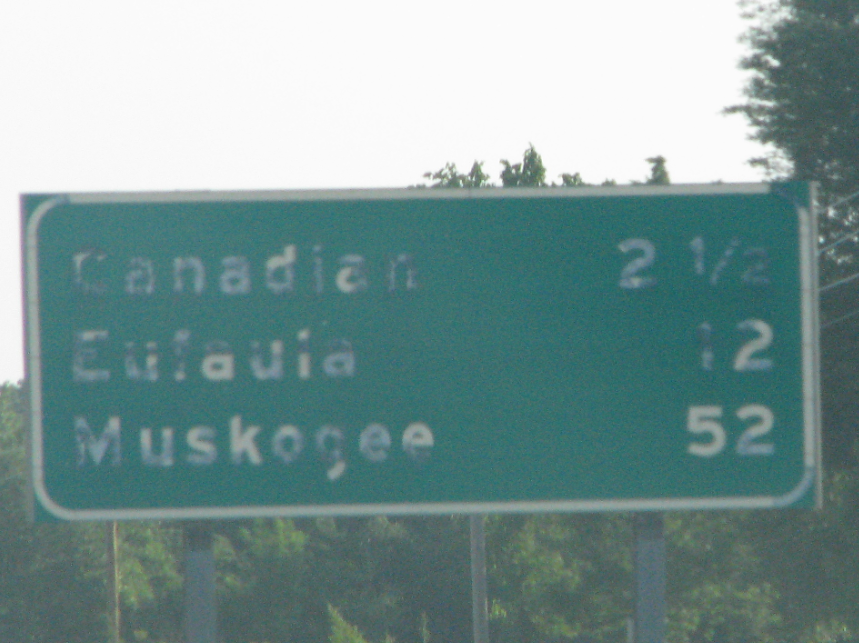This outdoor photograph captures a hazy sky at the upper part of the frame, with an array of trees spanning from the upper right to the lower left. The foliage varies in color, with patches of dark and light green where sunlight filters through. Power lines intersect the image, running in front of the trees. Prominently in the foreground is a rectangular sign, supported by two metal poles. The sign features a white rectangular border and white text that reads "Canadian 2 1⁄2," with an indiscernible word and the number "12" below it, and "Muskogee 52" at the bottom.